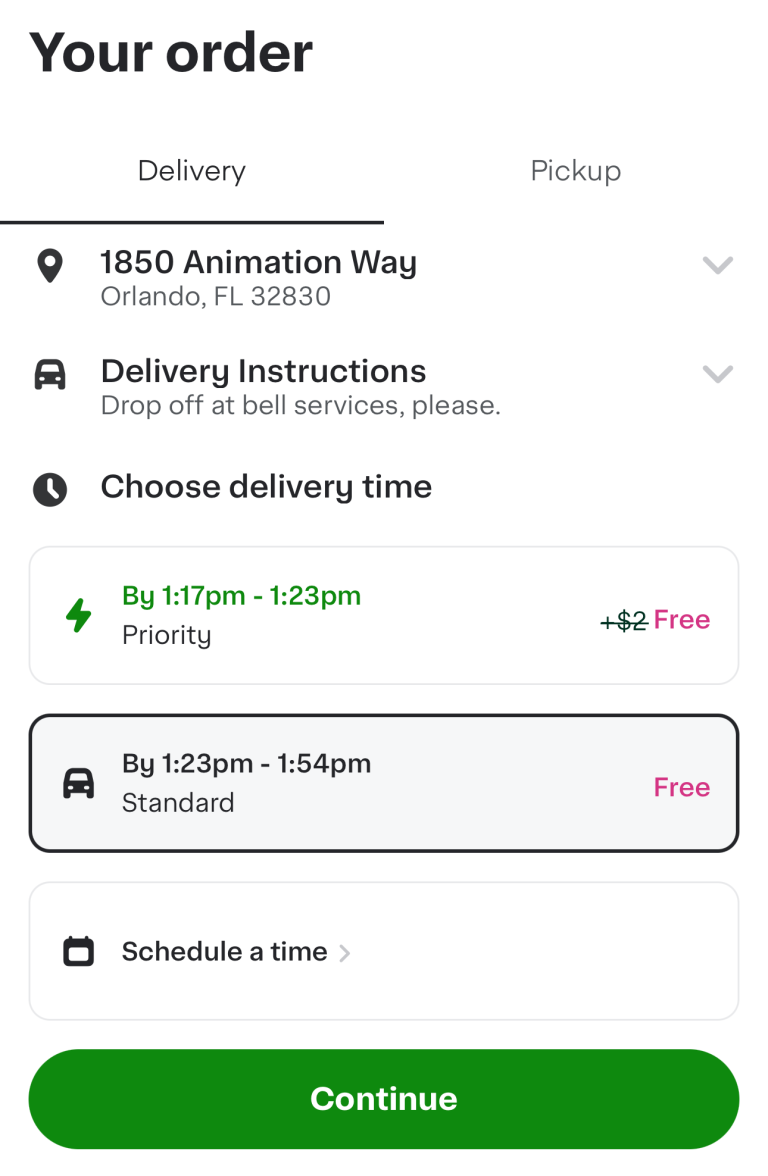This screenshot captures details of an online order page against a white background, blending seamlessly with the current webpage layout. At the top, bold black letters state, "Your Order." Below, there are two selectable options: "Delivery" and "Pick Up," with "Delivery" highlighted. 

Immediately underneath, there is a location icon followed by the address "1850 Animation Way, Orlando, FL 32830" with a dropdown arrow to its right. 

Further down on the left, an icon representing a car is displayed alongside the text, "Delivery Instructions: Drop off at Bell Services, please," with another dropdown arrow to its right. 

A clock icon appears below, accompanied by the option, "Choose delivery time." Beneath this, a highlighted box features green text indicating a priority delivery window: "By 1:17 PM to 1:23 PM," marked with a green lightning bolt icon. To the right of this, a plus sign and a "$2" charge (crossed out) appear, indicating a free delivery in pink letters. The selected box is slightly grayed out, detailing the standard delivery time: "By 1:23 PM to 1:54 PM," also marked as free in pink letters. 

Below this, another unselected white box features a calendar icon labeled, "Schedule a time," with an arrow pointing to the right. 

Finally, a green "Continue" button is positioned at the bottom of the screen.